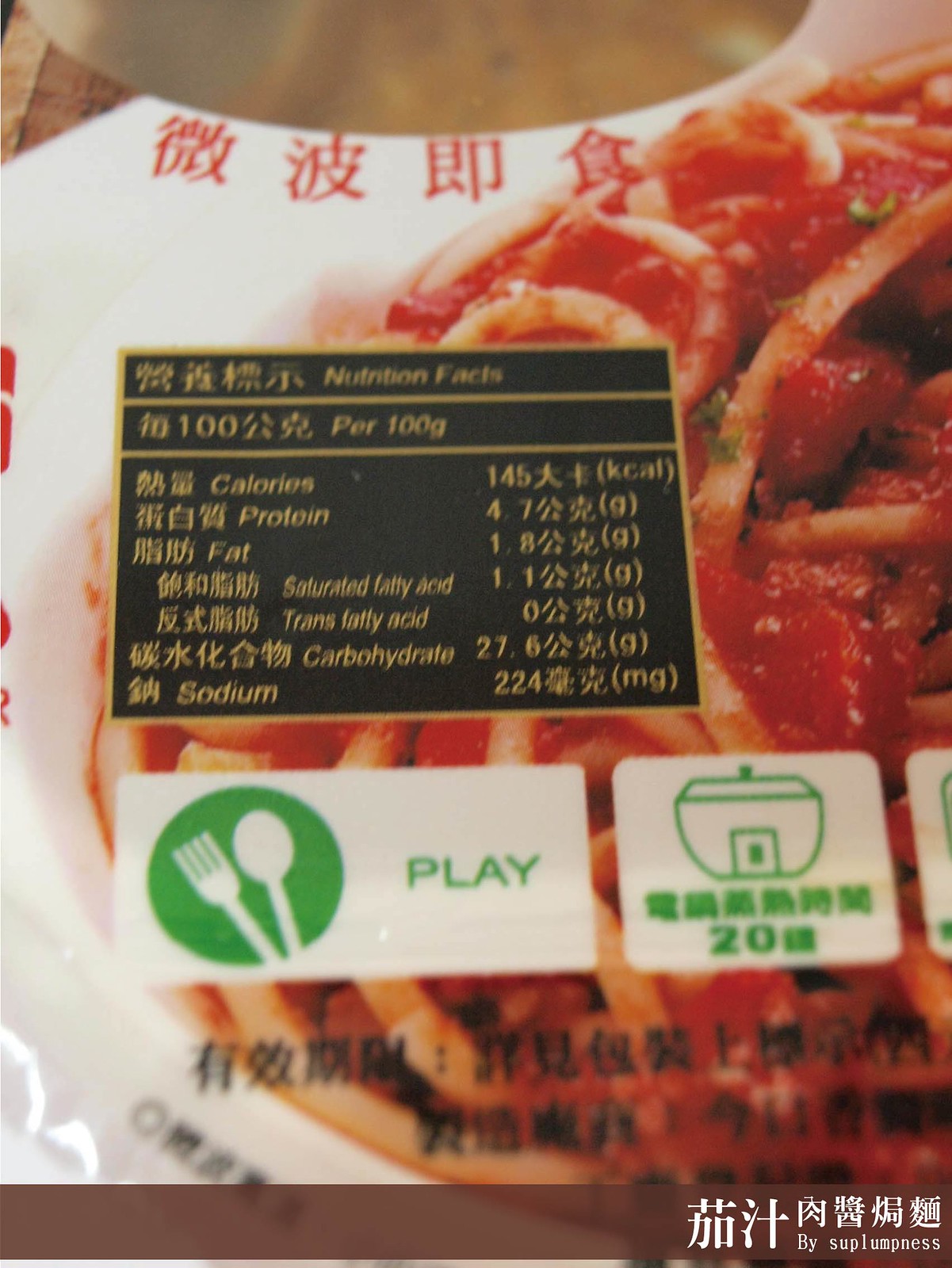This image is a vertically-oriented photograph of the back side of a packaged meal, likely of Asian origin given the abundance of Chinese or Japanese text. The packaging prominently features a photo of spaghetti. Central to the image is a nutrition label, enclosed in a black box with an orange border, listing nutritional information per 100 grams, including calories, protein, fat, saturated fatty acid, trans-fatty acids, carbohydrates, and sodium. Below this nutrition label, there is a white box with a green circle containing an illustration of a white fork and spoon, accompanied by the word "Play" written in green. To the right of this, there is another white box with a green-outlined device next to some Chinese text, which includes the number 20.